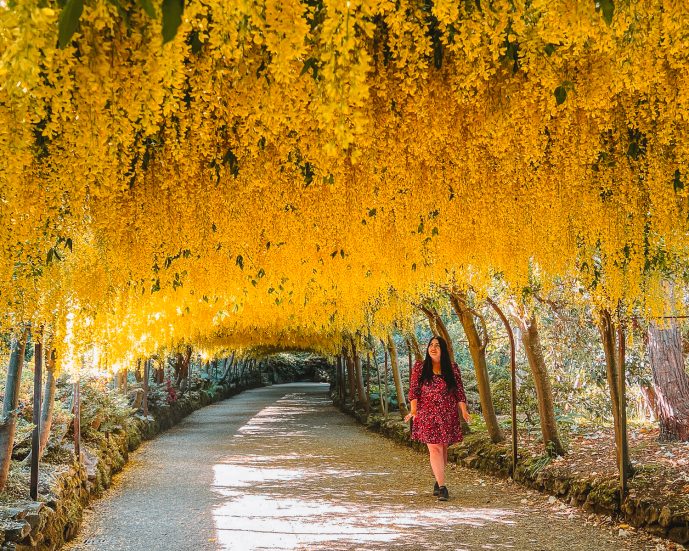In this vibrant, full-color photograph, a young woman with long dark hair and black shoes is captured walking down a wide, curving path made of cement, flanked by raised edges around a foot high and adorned with vegetation and rocks. She wears a striking red print dress and is visibly captivated by her surroundings, as she gazes upward with admiration. The scene is bathed in natural sunlight, speckling through the canopy of bright yellow flowering plants that arch over the path from trees on either side, creating a tunnel-like effect. The sun filters predominantly from the left side, casting playful shadows along the walkway. The lush, golden foliage, interspersed with glimpses of green leaves, completely envelopes the sky above, enhancing the sense of an enchanting, secluded retreat. In the background and to the right, tree trunks and additional greenery add depth to this picturesque, sunlit scene, highlighting the serenity and beauty of this outdoor haven.